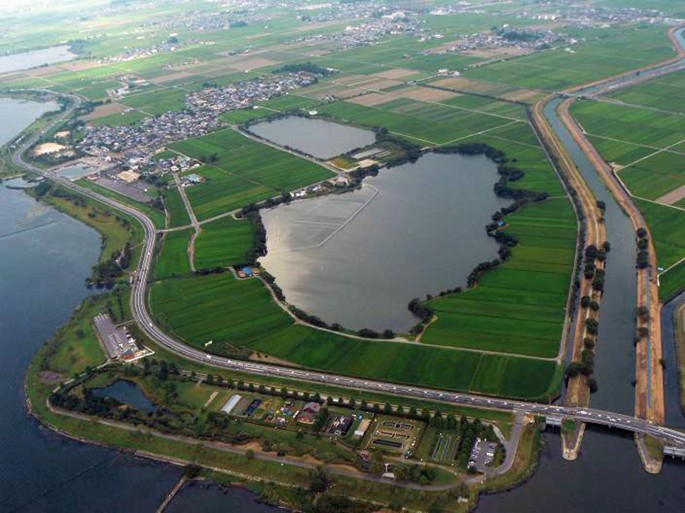This aerial angled view captures a scenic landscape next to a waterway, illustrating a harmonious blend of natural and urban elements. Dominating the center is a large lake encircled by lush green fields, indicating a possible farming region. The fields extend into various directions, interspersed with clusters of trees and perhaps a few baseball diamonds. To the left, a thin waterway wraps around the land and extends out into a larger body of water, encircling the area on the left and connecting with the lake through a river. In the bottom left corner, long docks jut out into the water next to a road that crosses a bridge, leading over the waterway. Upper portions of the image reveal densely packed neighborhoods, particularly in the upper left, while the upper right showcases more expansive green fields. Scattered houses and bustling roads with numerous cars weave through the landscape. Daylight bathes the whole scene, highlighting the vibrant greenery and the populated town that sits comfortably within this watery embrace.